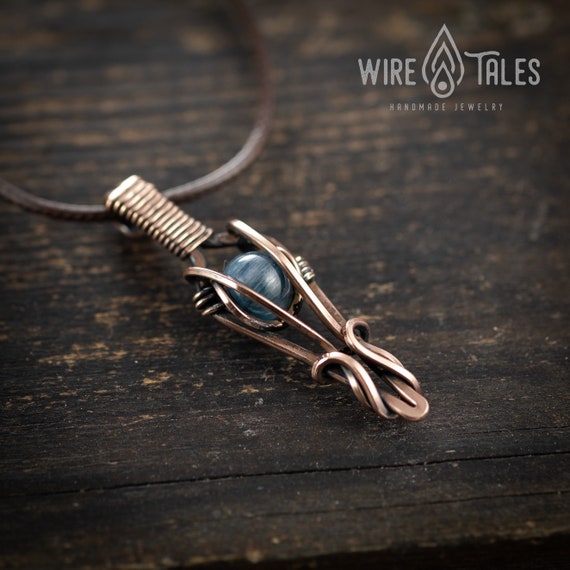This image showcases an intricately designed necklace laying on a worn, brown-painted wooden table, with patches of lighter wood showing through. In the top right corner, "Wire Tails" is written in light gray letters, accompanied by a small teardrop emblem, with the words "handmade jewelry" underneath in smaller text. The necklace features a brown leather or metal cord, which supports an elongated, tarnished gold pendant composed of segmented stripes. At the center of the pendant is a blue stone, resembling a marble, encased in a delicate cage-like structure made of wire, which securely holds the stone in place. The overall design is striking yet robust, blending feminine elegance with a touch of rustic charm.